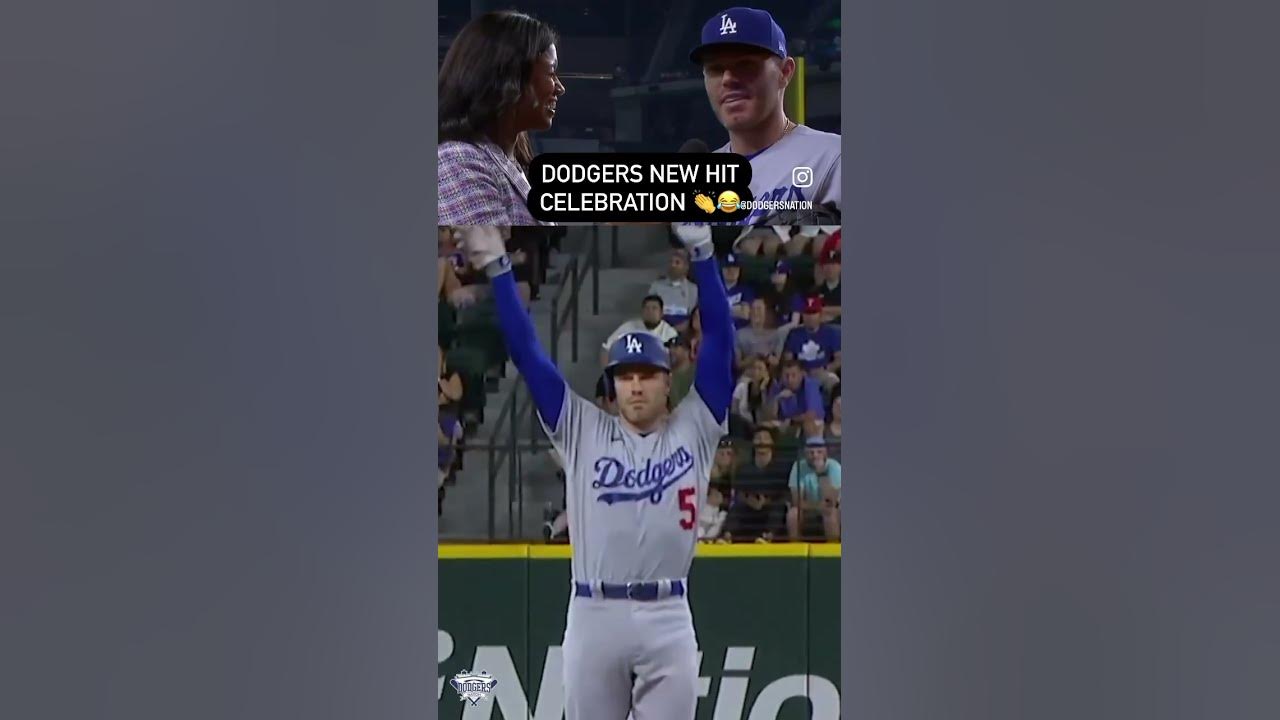The image is a vertically-oriented screenshot from an Instagram story, divided into two parts. The top third shows a joyful interaction between a smiling woman and a Los Angeles Dodgers baseball player wearing a blue cap with the white "LA" logo. Below this, in white capitalized text over a black background, is the caption "DODGERS NEW HIT CELEBRATION," accompanied by a clapping emoji and a crying-laughing emoji. The Instagram logo and the handle "@dodgersnation" are also visible in this section. The bottom two-thirds of the image feature the same baseball player, identifiable by his gray Dodgers jersey with the cursive "Dodgers" across the chest and the number 5 below it. He's celebrating with his hands raised, dressed in matching gray pants and a black belt. He appears to be in the midst of a game, with the shot showing him up to his knees.